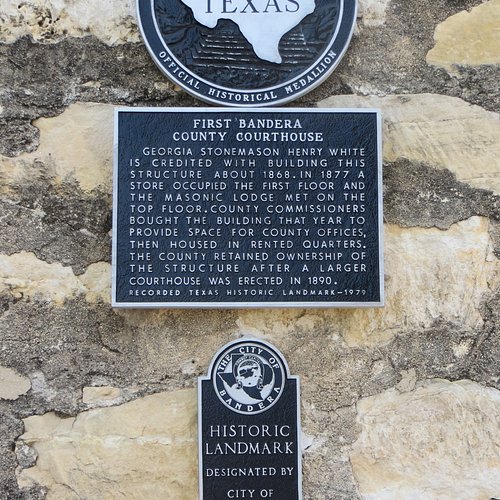The image depicts a historic landmark located in Texas, specifically the First Bandera County Courthouse. The scene centers on a rough, tannish-white stone wall with gray grout, presumably part of the historic courthouse structure itself. Affixed to this wall is a series of plaques. At the top, partially visible, is a circular medallion featuring an image of Texas labeled "Texas" and denoting its official historical status. Below this medallion is a rectangular plaque detailing the courthouse's history, noting that it was constructed by Georgian stonemason Henry White around 1868. It further explains that in 1877, the building's first floor housed a store while the Masonic Lodge used the top floor. That same year, county commissioners purchased the building for county office space, maintaining ownership even after a larger courthouse was built in 1890. This building has been recorded as a Texas Historic Landmark since 1979. Beneath the historical text plaque, there is another smaller circular plaque with the words "The City of Bandera" around the rim and an image of Texas in the center, likely signifying the historic designation by Bandera city authorities. The plaques are characterized by dark charcoal gray with silver writing, contrasting against the lighter stone wall.